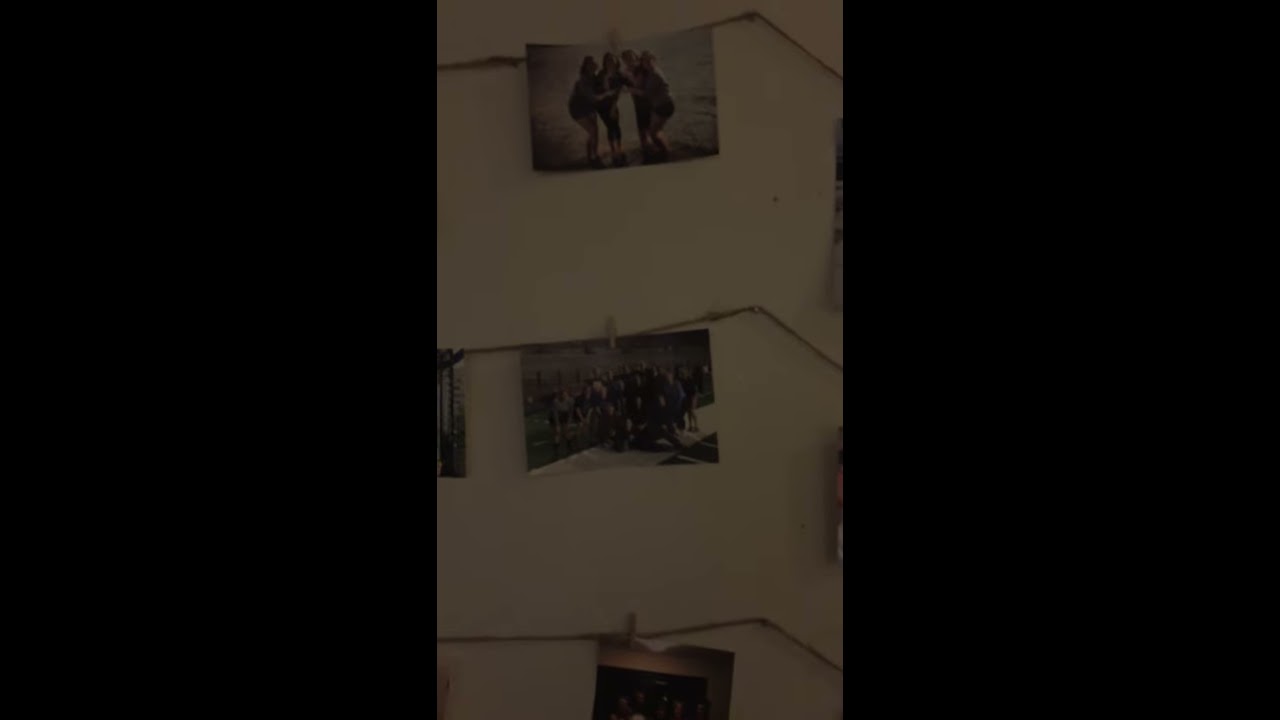The image depicts a white wall adorned with three rows of brown string, each string secured to the wall with nails and featuring photographs clipped on with what appears to be clothespins. The topmost photograph shows four women by a body of water, either standing or kneeling and looking at the camera. The middle row contains a photo of a large group of people, potentially indicating a sports team or a social gathering. The lowest photograph remains indistinguishable due to brightness. The display evokes a nostalgic, old-fashioned charm, reminiscent of the 1990s and suggests a setting that could be a bedroom, office, or another personal space.